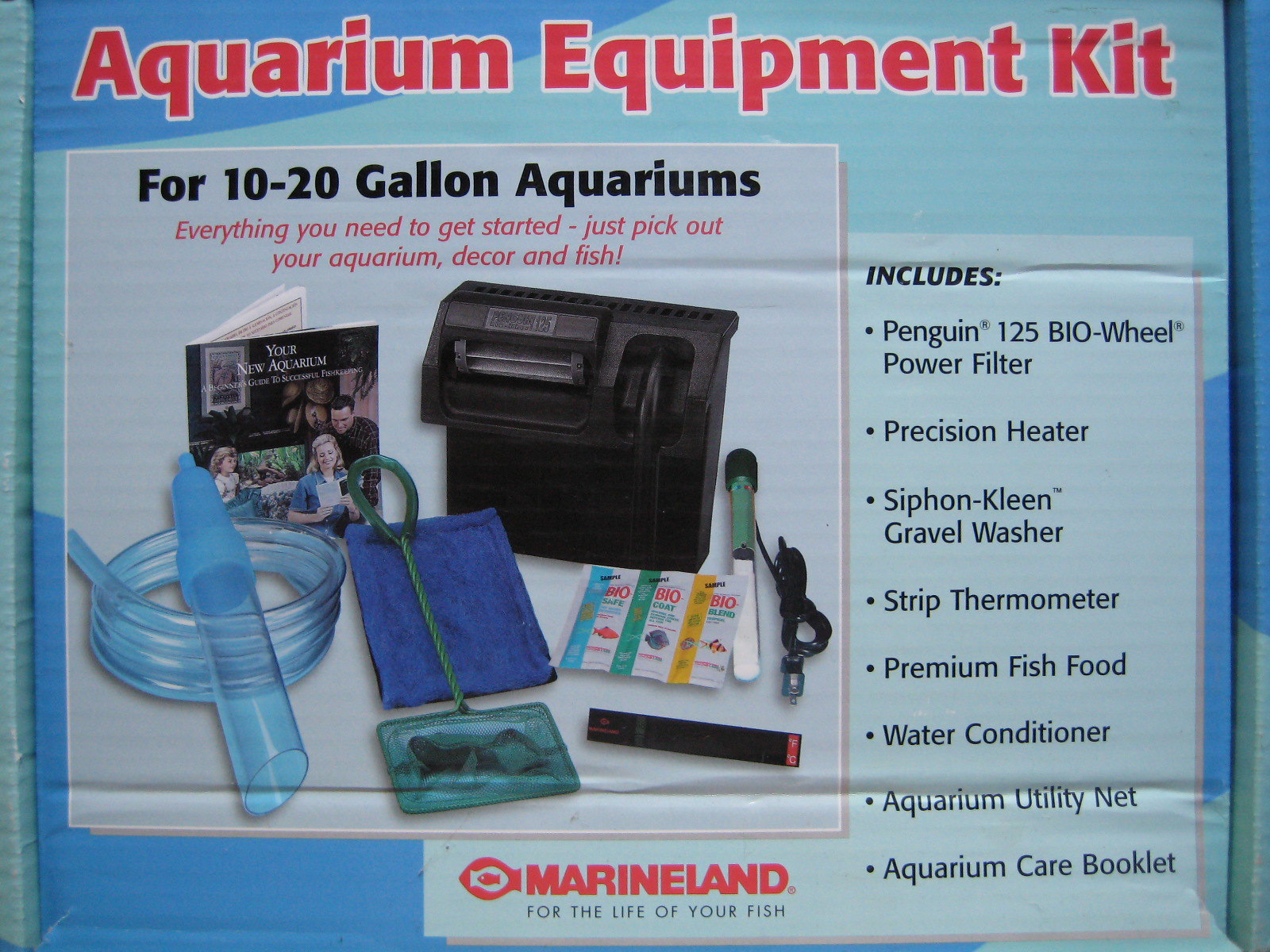The image shows the side of a rectangular boxed aquarium equipment kit, primarily set against a dark blue background with light blue accents. Prominently displayed at the top in bright red font outlined in white, it reads "Aquarium Equipment Kit." Below this, the box indicates suitability for 10-20 gallon aquariums in black text. The package highlights that it includes everything needed to get started, with the phrase "everything you need to get started" also in red. The front of the box features images of the kit's contents, which include a piece of tubing, a net, a black filter, packets of food, and a booklet. Additional items listed are a filter, heater, strip thermometer, water conditioner, and food. The company's name, Marine Land, is displayed at the bottom in red, accompanied by a fish logo and the tagline "for the life of your fish."